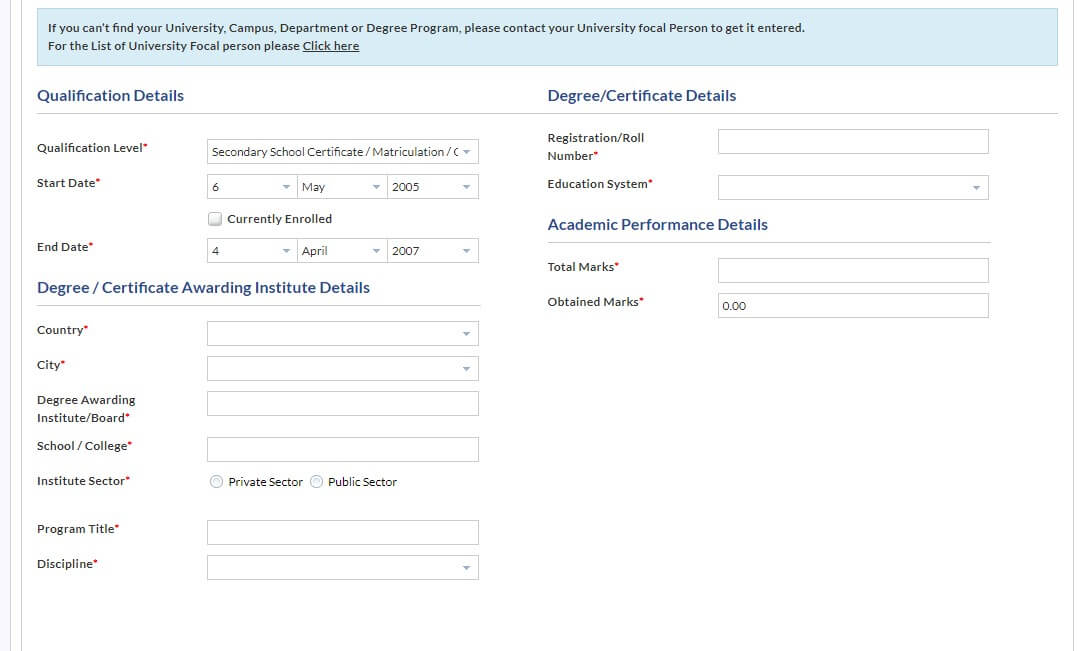If you are unable to find your specific university, campus, department, or degree program, we recommend contacting your university directly to resolve the issue. For a comprehensive list of universities, please click here. The necessary qualification details include Degree Certificate Details, Qualification Level, Start Date, End Date, Registration and Role Number, Education System, and Academic Performance Details such as Total Marks and Obtained Marks. You will also need information on the Degree/Certificate Awarding Institute, including the Country and City of the Awarding Institute/Board, School/College, Institute, and the designation of the Sector (Private or Public). Furthermore, make sure to provide the Program Title and Discipline associated with your degree.

[Include relevant link for “click here”]